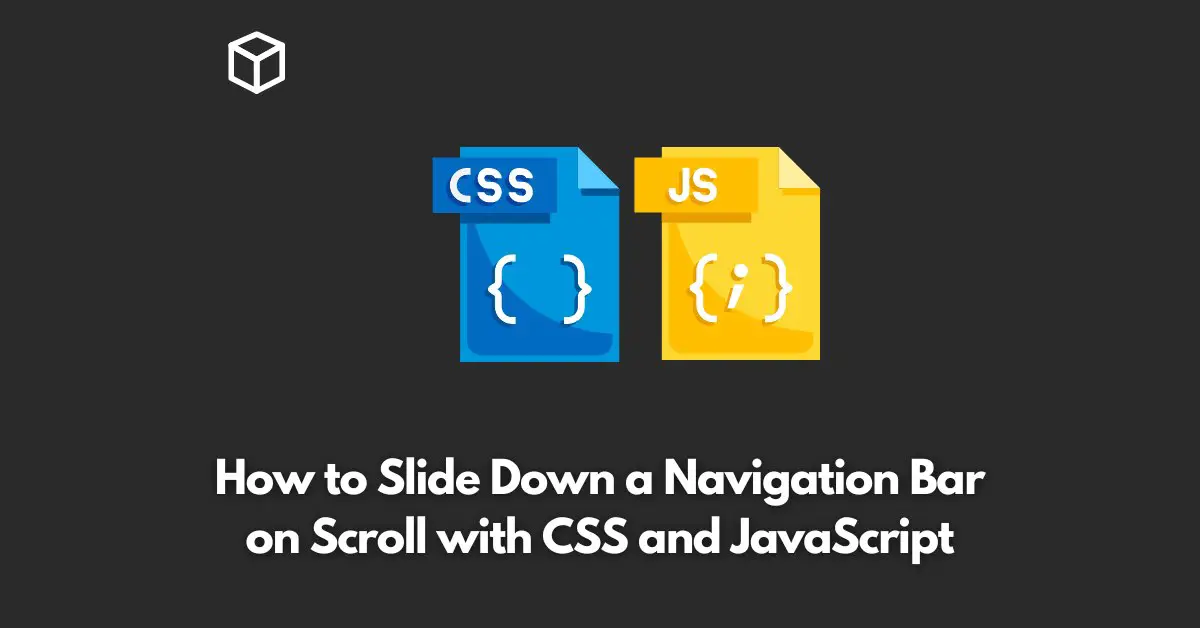The image features a dark grey background with a prominent white isometric drawing of a cube at its center. The cube, resembling the familiar three-dimensional form, is depicted using three diamond shapes joined together, showcasing two visible facets and the top surface.

To the left of the cube, there is a blue document icon with a folded corner. The icon displays a pair of brackets with a small blue overlay panel containing the text "CSS" in a darker shade. On the right side, another document icon mirrors the design but is colored yellow. This icon also has brackets, along with an 'eye' symbol between them, and features the text "JS" on a darker yellow overlay. Both document icons exhibit a shading effect at their lower left corners, giving them a somewhat three-dimensional appearance.

Below these icons, there are two lines of bold white text. The first line reads "How to Slide Down a Navigation Bar" and the second line says "Unscroll with CSS and JavaScript." This suggests the image is part of an instructional guide on how to create a sliding navigation bar using both CSS and JavaScript.